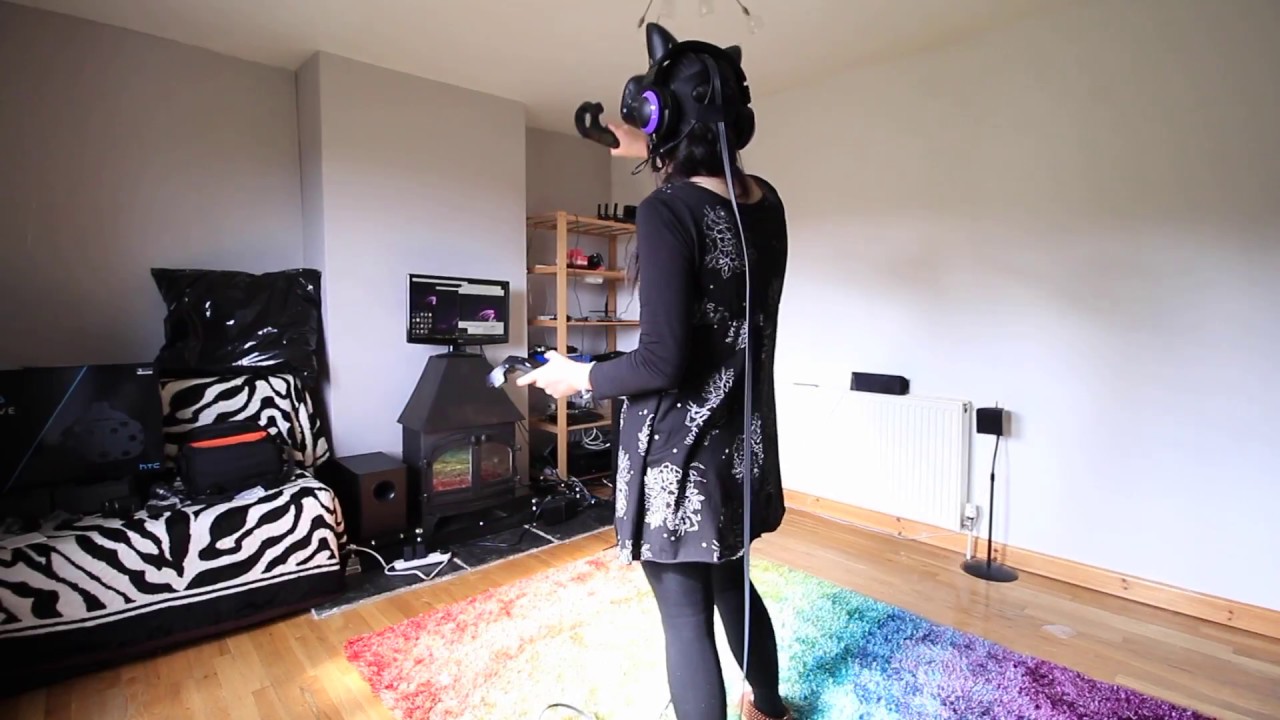In this detailed image, we see a woman engaged in a virtual reality game, standing prominently in the center of a living room. She is a white female, dressed in a long black dress with white accents, paired with a long-sleeved black t-shirt and black leggings that extend to her feet. Over her head, she wears a virtual reality headset adorned with cat ears and purple earmuffs, obscuring her eyes. She holds a black controller in each hand, with cords trailing from the headset to the floor, indicating her immersion in the VR experience. 

The living room setting encompasses a mix of modern and eclectic decor: the walls are painted a grayish white, and the natural hardwood floor is partly covered by a vibrant area rug featuring shades of purple, blue, light blue, and potentially other colors forming a rainbow-like pattern. Against the far wall stands an eye-catching zebra-patterned couch, accompanied by a small fireplace, a TV, a bookshelf loaded with books, and a radiator heater on the right side. The baseboards frame the room, adding a subtle architectural detail to the overall setup.